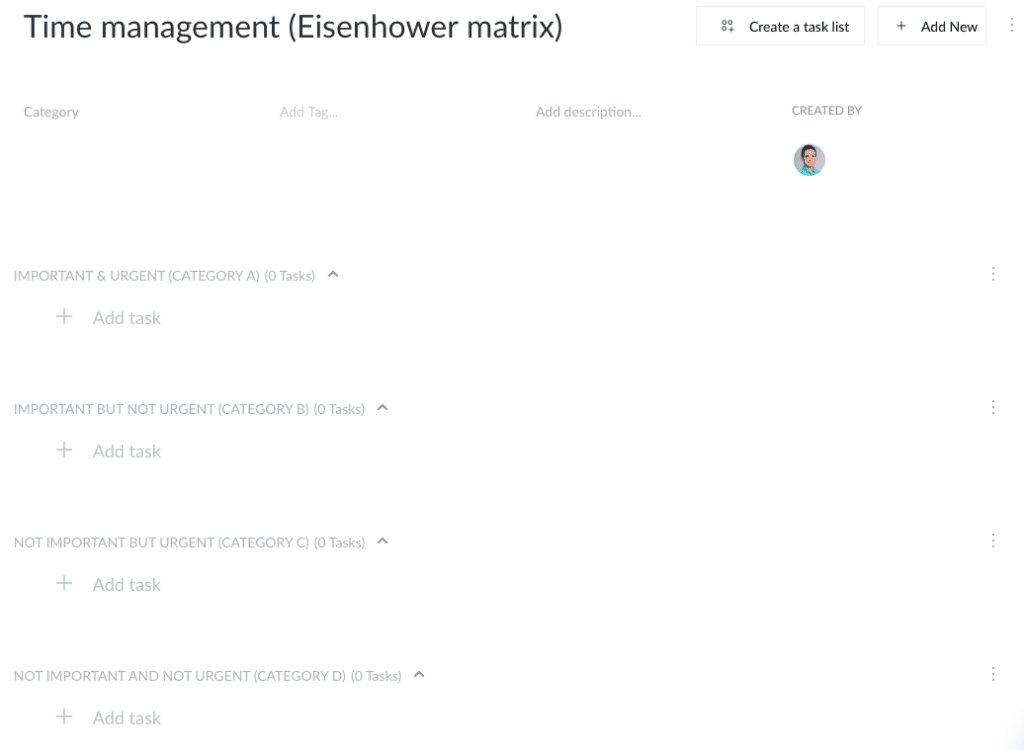Screenshot Description: Eisenhower Matrix Layout

The screenshot displays an application screen titled "Time Management (Eisenhower Matrix)" at the top in black text. On the right side of this top bar, there’s an option labeled "Create a task list" accompanied by a "+ Add New" button and a submenu denoted by three gray dots.

Below the title, the screen is segmented into the following sections, all of which are grayed out, indicating no interaction has occurred:

1. **Category Management Section:**
   - **Category, Add Tag, Add Description:** 
     Each option appears in gray text.
   - **Created By:** 
     Beside this, there is a circular avatar icon that is unselected, presumably representing a user.

2. **Task Management Sections:**
   - **Important and Urgent (Category A):**
     - Displays "0 tasks" in gray text.
     - Includes an up arrow next to "0 tasks" (likely to collapse the section).
     - "+ Add Task" button is visible.

   - **Important, but Not Urgent (Category B):**
     - Displays "0 tasks" in gray text.
     - Features an up arrow next to "0 tasks."
     - "+ Add Task" button is present.

   - **Not Important, but Urgent (Category C):**
     - Displays "0 tasks" in gray text.
     - Contains an up arrow next to "0 tasks."
     - "+ Add Task" button is included.

   - **Not Important and Not Urgent (Category D):**
     - Displays "0 tasks" in gray text.
     - Contains an up arrow next to "0 tasks."
     - "+ Add Task" button is present.

Given the entire section is grayed out, it suggests that the matrix has not been populated with data, and there might be limited or view-only access currently granted.